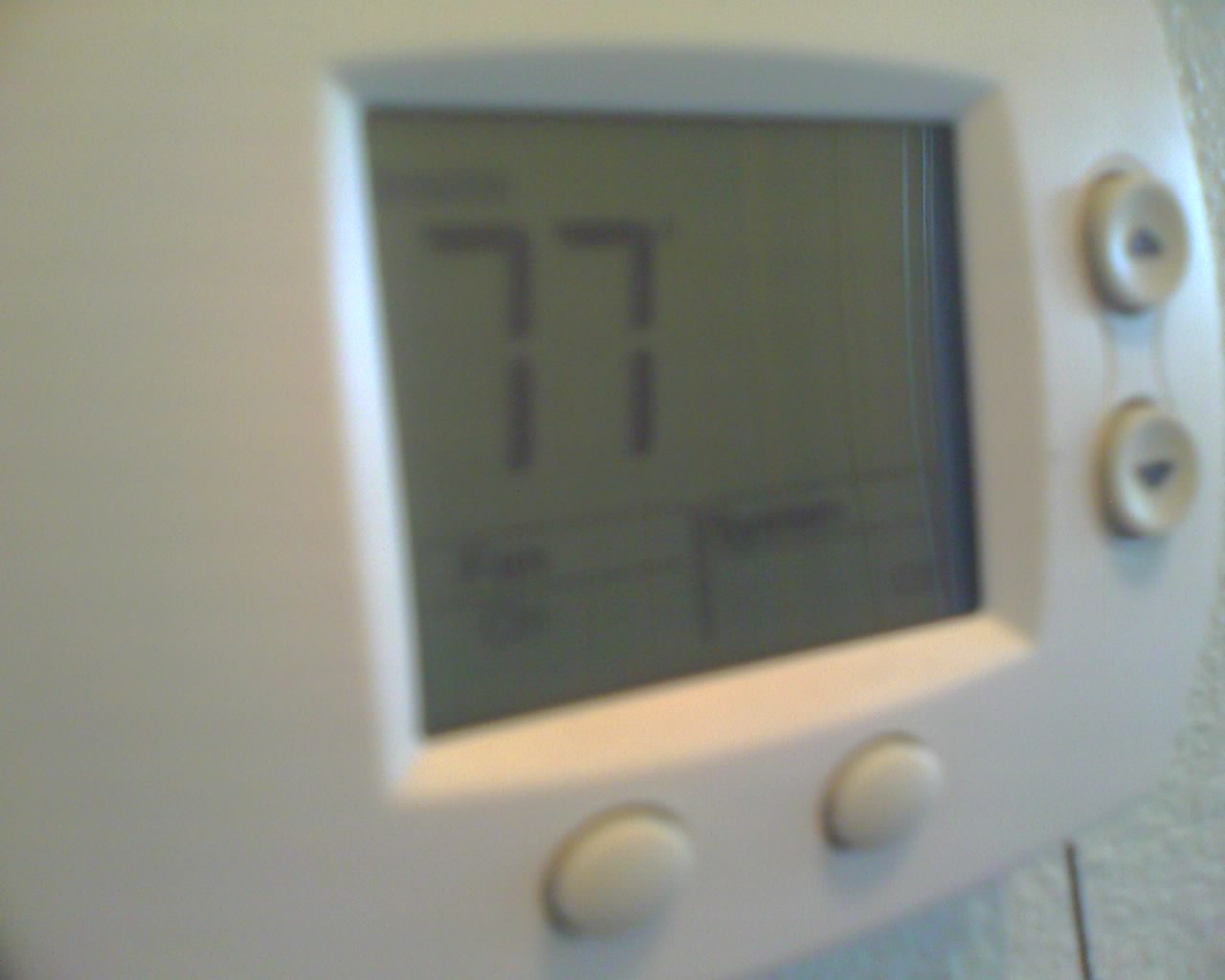This image features an extreme close-up of a digital thermostat, occupying almost the entire frame and cutting off parts of the device. The thermostat partially obstructs its own view, leaving the upper left corner and the left edge outside the image's bounds, while the right side displays a curved edge seamlessly transitioning to a flat bottom. The backdrop consists of a distinctively textured white wall, visible around the bottom right and top right corners.

Dominating the lower section of the image is a white plastic enclosure framing the digital screen. Two unmarked buttons reside at the bottom, while additional controls for fan speed adjustment are also present, indicating the ability to modify temperature settings directly. The display reads a current temperature of 77 degrees, with the word "fan" visible in a small box. Directly below, another box shows the label "off," suggesting options for easy functionality changes. The thermostat's design and interface imply user-friendliness, allowing for straightforward room temperature adjustments.